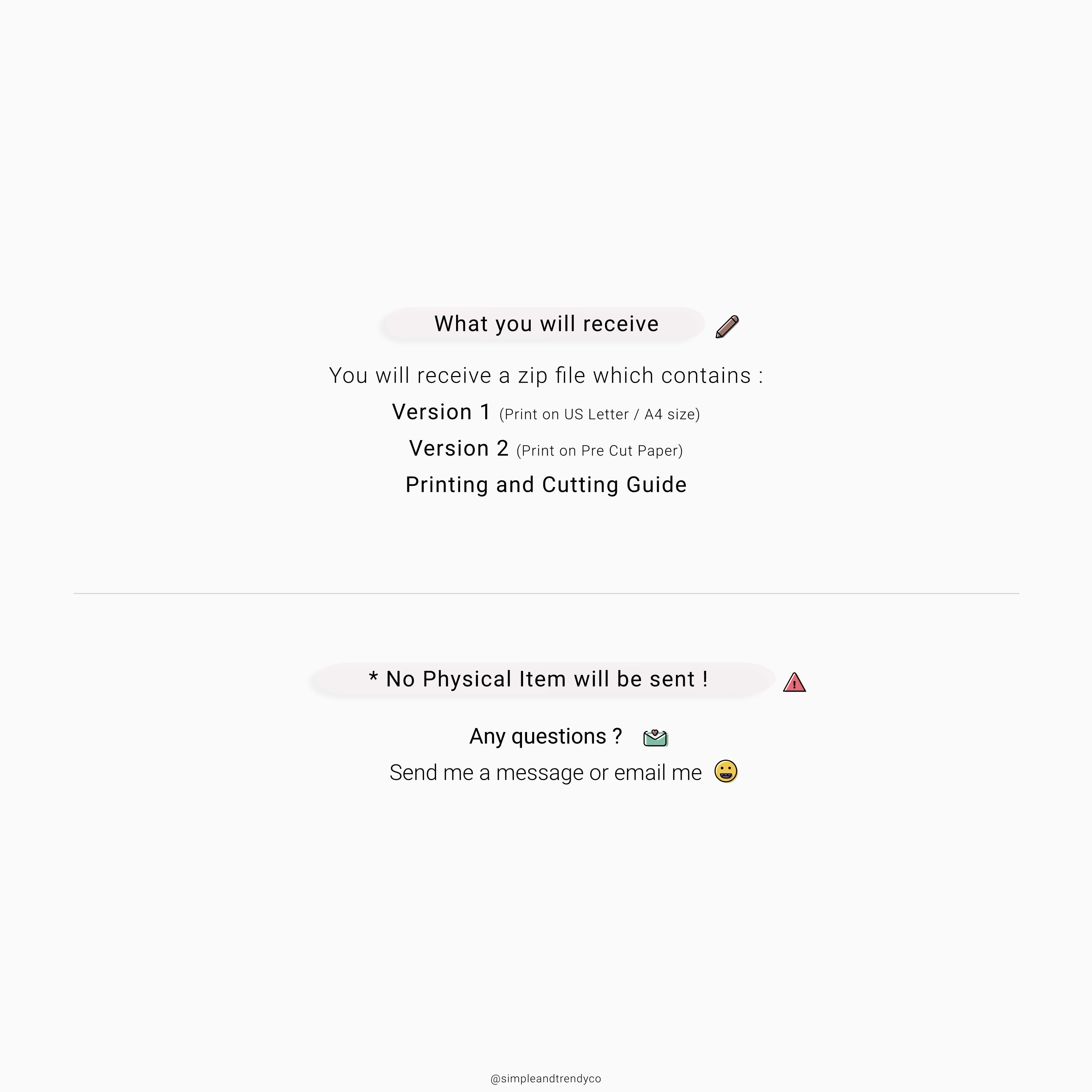This image depicts a screenshot with a black background featuring text in the center. The text is organized into different sections:

1. The top section, in larger, prominent font, reads, "What You Will Receive," followed by an icon resembling a pencil.
2. Below this header, it specifies the contents of a zip file: 
   - *Version 1*: Print on US Letter/A4 size.
   - *Version 2*: (Print on pre-cut paper)
   - Printing and Cutting Guide.

A faint gray line separates the next section.

3. The bottom section features a star icon and a warning in bold: "No physical item will be sent!," accompanied by a triangle with an exclamation mark inside.
4. It then prompts, "Any questions?" followed by an email icon.
5. The text encourages, "Send me a message or email me," and a yellow smiley face icon is present next to this statement.
6. At the very bottom of the image, there is small print text, though it is not clearly legible in the caption provided.